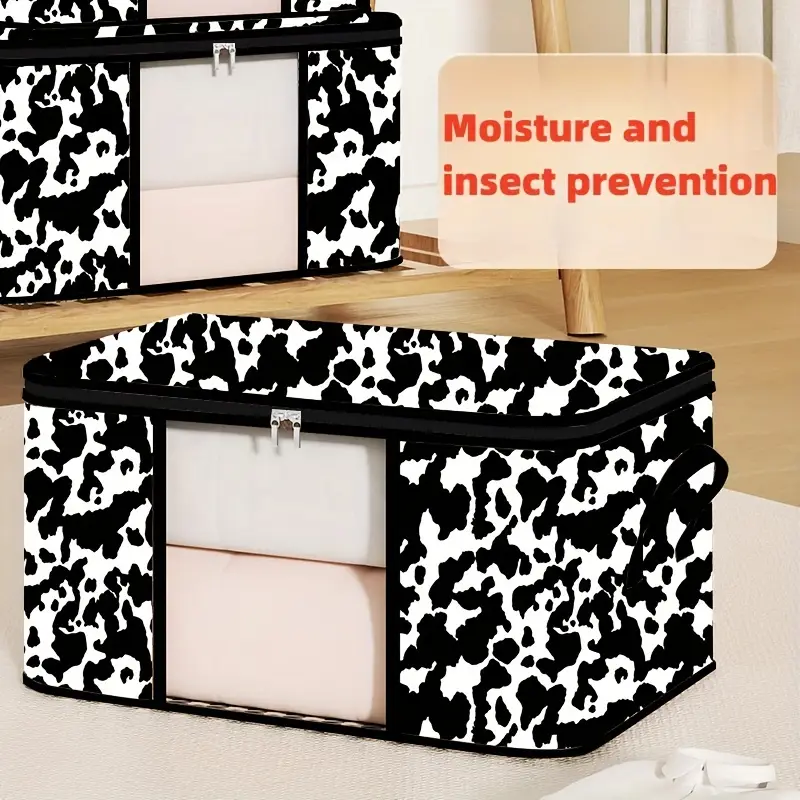The image depicts two black and white storage boxes, designed with a cow print pattern and prominently advertising their moisture and insect prevention capabilities. These boxes, which appear suitable for under-the-bed or closet storage, feature zipper closures that meet in the middle and open from both directions. A transparent panel on the front measures approximately 8 to 10 inches wide, allowing visibility of the contents within. Inside one of the boxes, pastel-colored blankets or sheets are visible through this clear panel. The boxes are positioned on a light wood surface, which could be either a table or a wood floor, and the one at the front is placed on a round, rubberized mat. In the background, there are drapes and a wooden pole, suggesting an indoor setting. The image notably includes a sign that reads "moisture and insect prevention," likely indicative of the boxes' features.